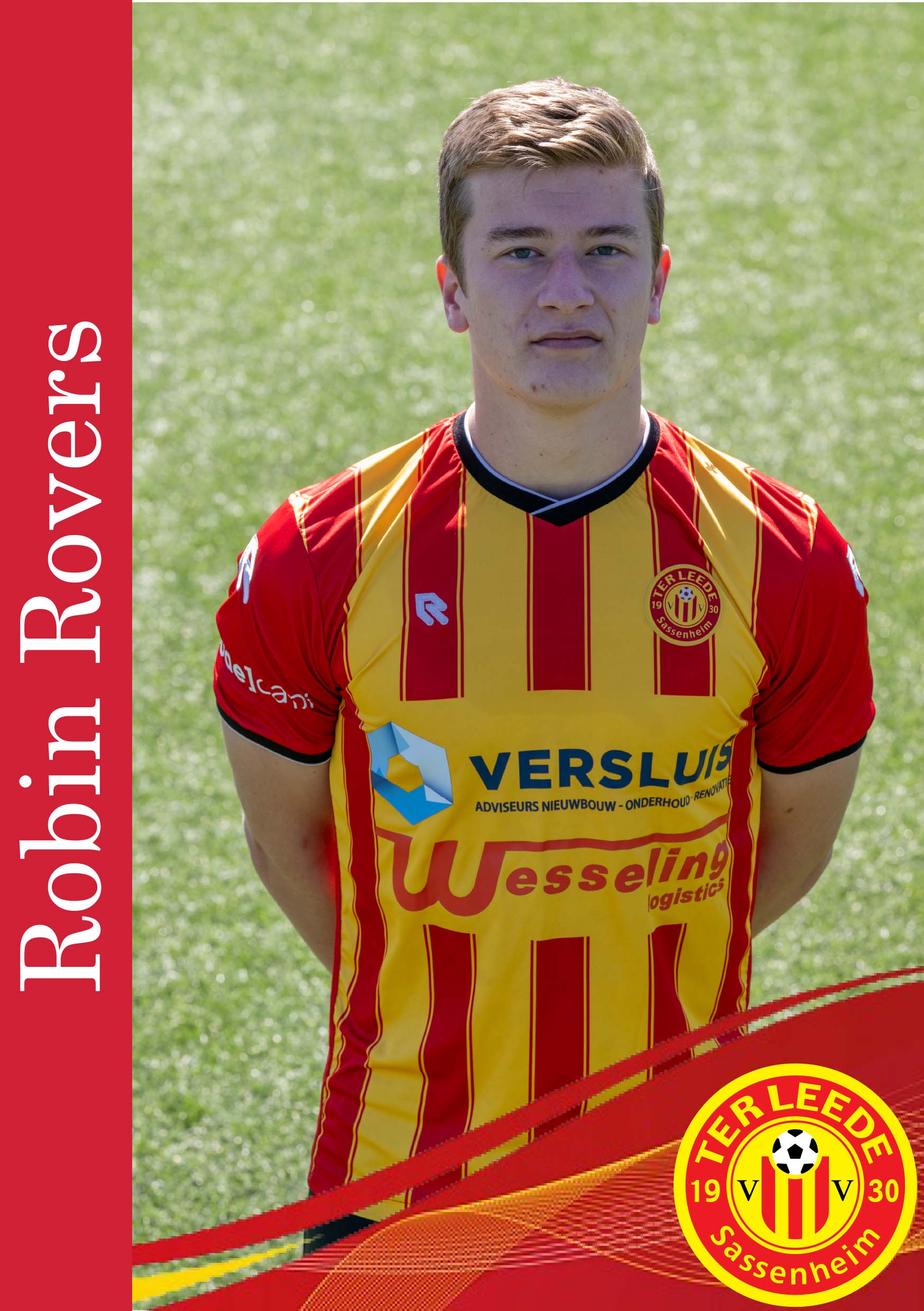The image depicts a young male soccer player with short blonde hair, possibly around 17 years old. He stands on a grassy field, facing the camera with a neutral expression, his hands clasped behind his back. He wears an orange, yellow, and red striped jersey prominently displaying "Versluthe Westling" across the center in blue and red lettering. The left side of the image features a red vertical banner with white text reading "Robin Rovers." On the player's left breast is an emblem containing a yellow circle with a soccer ball, bordered by red and yellow lines, inscribed with "Ter Leeds, 1930, Sassenheim." The background consists of the green grass field, lending a vibrant contrast to the player’s colorful jersey and the emblem. The overall composition, including a thin red border on the left side, suggests it could be a promotional card or magazine cover.